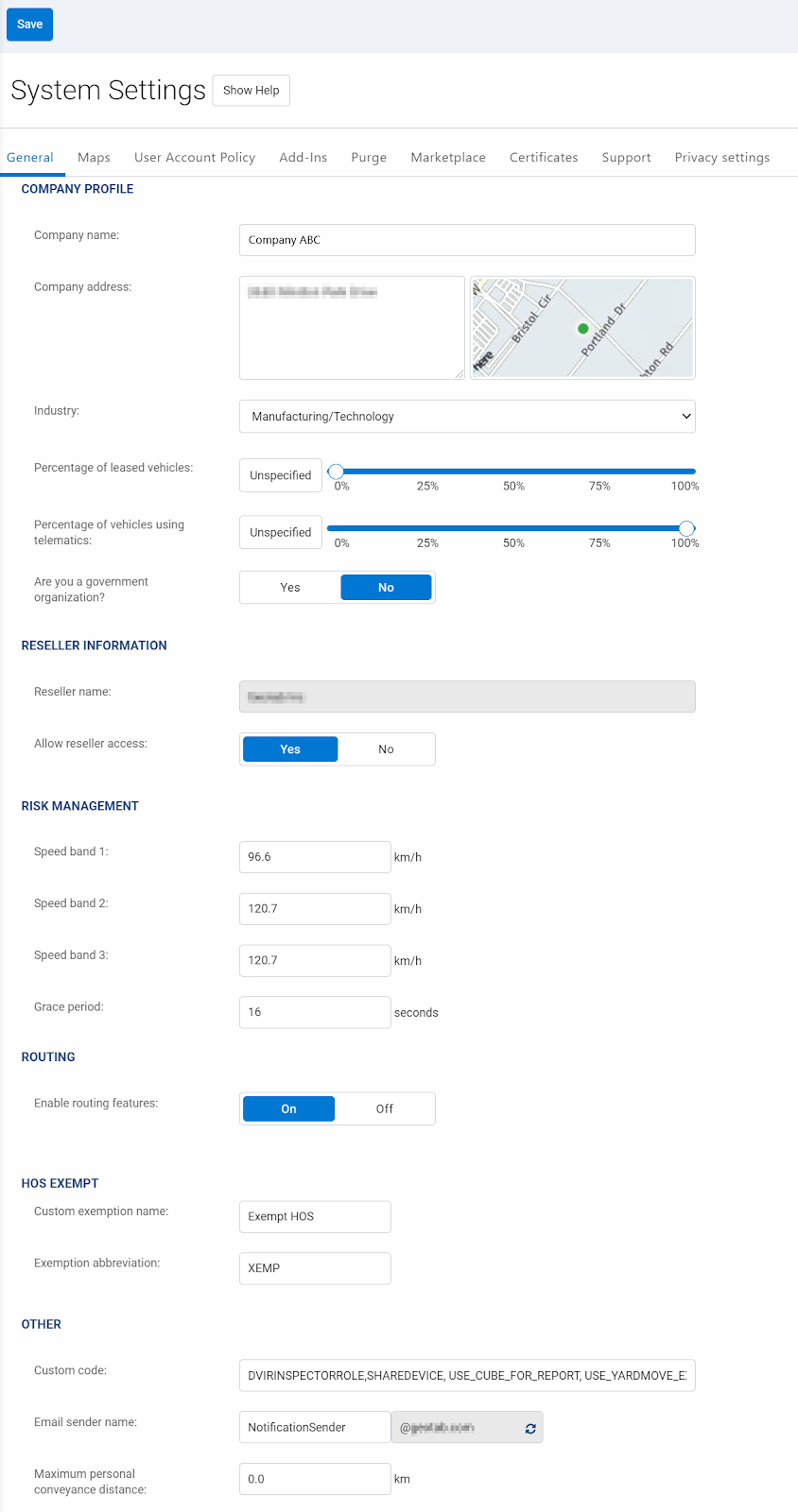This image showcases an informational window on a computing device, most likely a computer given the format and layout. Although the dialog box style is unfamiliar and not recognizable as Windows, certain details stand out. The small, black-on-white text near the top reads "System Settings." Directly beneath this title, the specifics are illegible due to the diminutive font size. Three blue buttons are visible, presumably interactive, though their functions are not discernible. There is also a light gray tile, possibly illustrating a segment of a map. Along the left side of the window, there is a menu featuring blue-titled categories with four or five gray options listed under each. Like the rest of the text, these options are too small to read clearly.